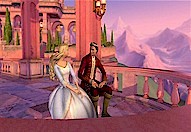A small, computer-generated image captures a regal scene resembling a video game screen cap. A prince and princess are seated on a balcony, exuding elegance and grace. The princess, with her flowing blonde hair, wears a stunning white dress featuring a voluminous, fluffy skirt. Beside her, the prince dons a luxurious red velvet suit paired with knee-high boots, epitomizing nobility.

The setting bathes in a captivating pinkish glow, suggesting the mellowness of a sunset. In the distance, a light purple mountain range stretches across the horizon under a sky painted in soft shades of pink and purple. The balcony flooring consists of purple tiles, and the space is adorned with pillars extending towards the back. The majestic building, characterized by its light pinkish hue and arched frames, stands as a testament to architectural splendor. Surrounding the structure, verdant green trees add a touch of natural beauty to the scene.